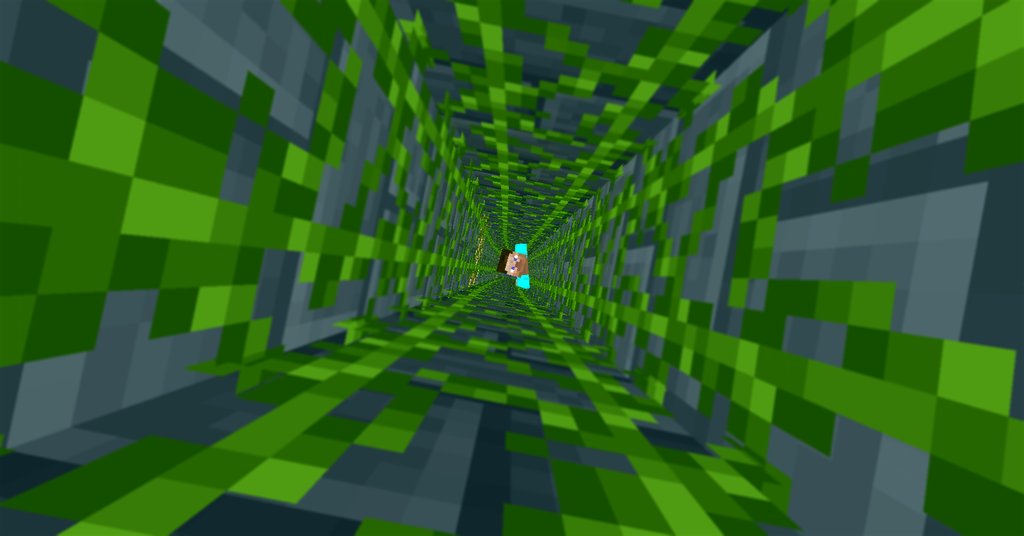The image is a screenshot from a game, likely Minecraft, depicting an optical illusion of a deep shaft or tunnel composed of various colored squares. The tunnel's sides feature a pattern of small squares in shades of dark green, medium green, light green—all with yellow undertones—along with dark gray, medium gray, and light gray. In the center of the image, there is a small, blocky figure with a brown face and dark hair, resembling a cartoon image of an African American man. He is dressed in what appears to be a turquoise shirt with two aqua squares on either side, representing shoulders. The figure seems to be descending or trapped in this endless square tunnel. There is no text, player information, or additional features in this screenshot, emphasizing the depth and the character's position within the intricate, colorful shaft.